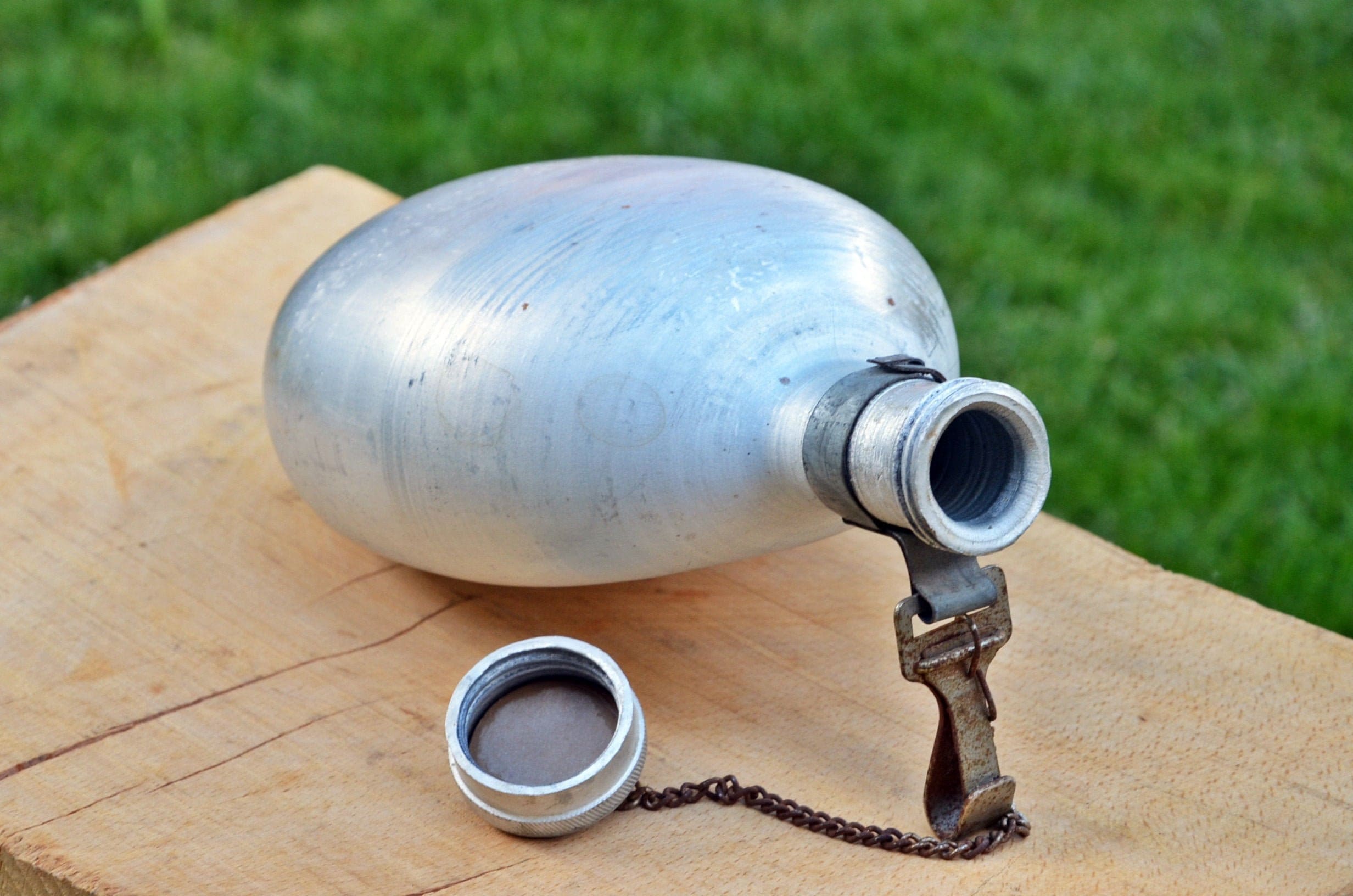The image features a small, high-quality stainless steel canteen with a light silver brushed metal finish, resting on a rectangular wooden surface with visible horizontal striations and four vertical cracks. The canteen, possibly used for water or even gunpowder, is compact enough to fit in the palm of your hand. It has a robust construction with no risk of leaks or cracking. Its stainless steel cap, which is detached and positioned beside it, is connected by a thin, rusty brown chain. The canteen is stabilized at a 90-degree angle by a clasp device underneath it. The backdrop of the image consists of vibrant green grass, which appears blurry.